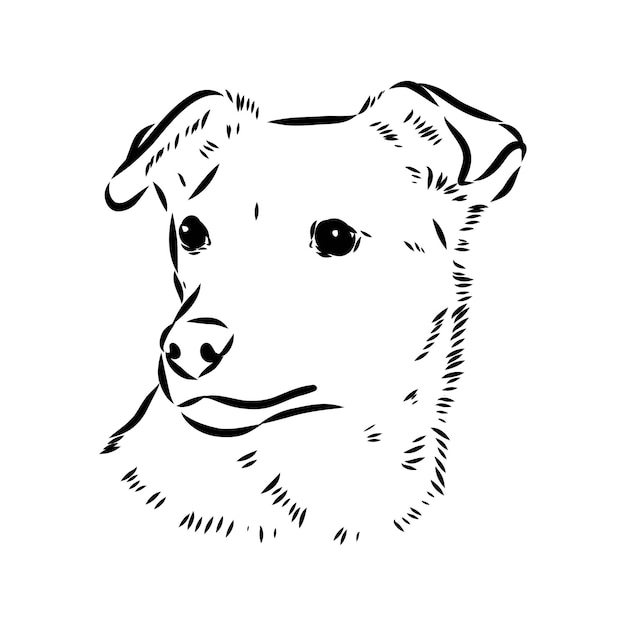The image features a minimalist, black-and-white sketch of a dog set against a completely white background. The dog is depicted from the top of its head down to its neck, with its ears flapping down and eyes looking to the left, as if something has caught its attention. The illustration captures details such as the dog's black eyes with white dots, its nose, and mouth. Thin, short lines adorn the dog's outline to suggest fur texture, adding to its appearance of a collie or possibly an Australian Shepherd. The headshot emphasizes the dog's eyes, nose, and fur detailing, without any signature or indication of the artist.